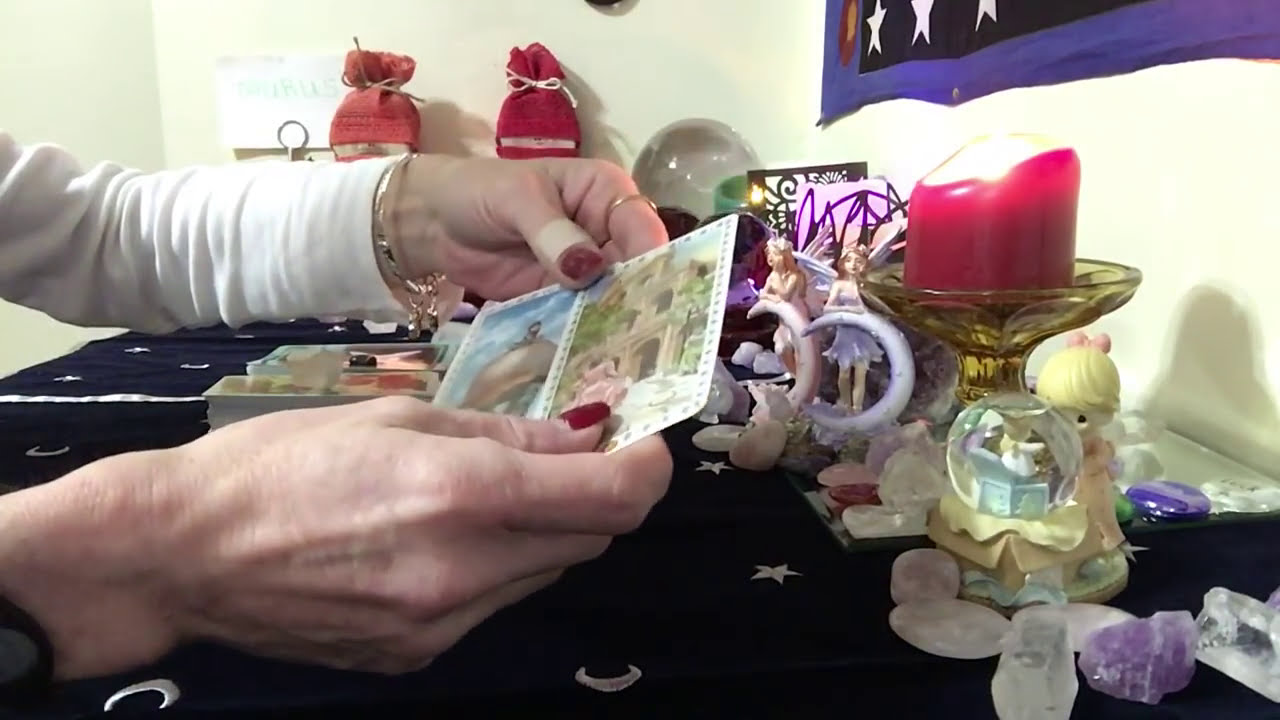A detailed close-up image showcases a pair of Caucasian female hands holding what appears to be a set of tarot or oracle cards. The hands, with nails meticulously painted in a dark red polish, are adorned with a gold ring on the left index finger and a black watch on the right wrist. Notably, the left thumb sports a band-aid, and a gold bracelet with dangly pendants graces the wrist. The hands are positioned over a dark velvety tablecloth, decorated with white stars and quarter moons, suggestive of a mystical or spiritual setting. The table, which likely functions as an altar, is scattered with an assortment of crystals, gems, and figurines, including fairies and a red candle in a glass holder. The background features a white wall adorned with a purple-bordered tapestry, adding to the mystical ambiance. In the upper left corner, two red hats are visible, contributing an additional pop of color to the scene.